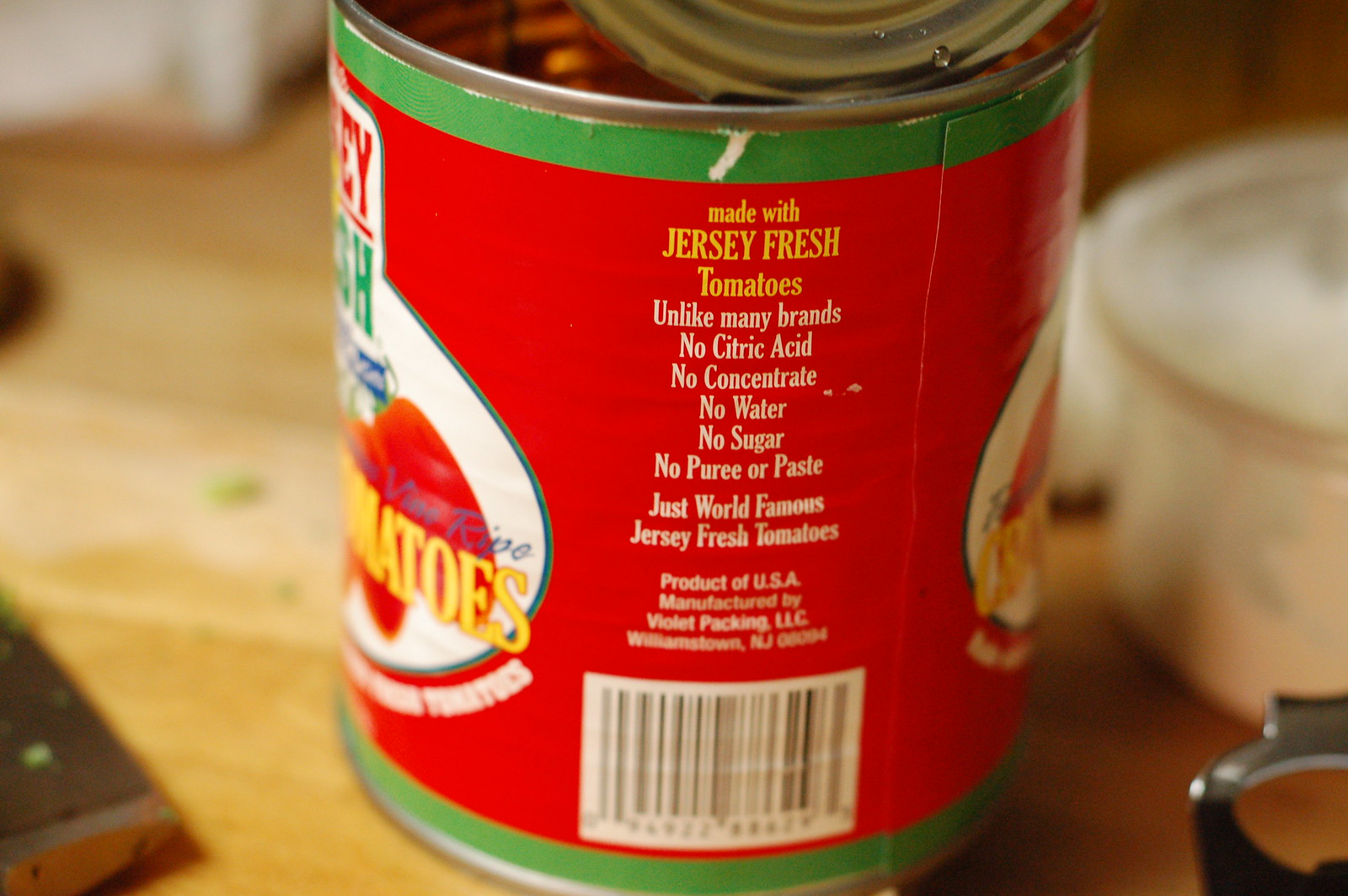The image features an opened can of tomatoes prominently displayed on a wooden kitchen counter. The can's label, which is predominantly red with green trim around the top and bottom, is partially visible. The text on the visible side of the label reads: "Made with Jersey Fresh Tomatoes. Unlike many brands, no citric acid, no concentrate, no water, no sugar, no puree or paste. Just world-famous Jersey Fresh tomatoes. Product of USA. Manufactured by Violet Packaging LLC, Williamstown, New Jersey." A barcode is also visible beneath this text. Although the front of the label isn't directly shown, it can be inferred that it says "Vine Ripe Tomatoes." In the background on the right side of the image, a pot is slightly visible, adding context to the kitchen setting. The primary focus remains on the can of tomatoes, emphasizing its quality and origin.